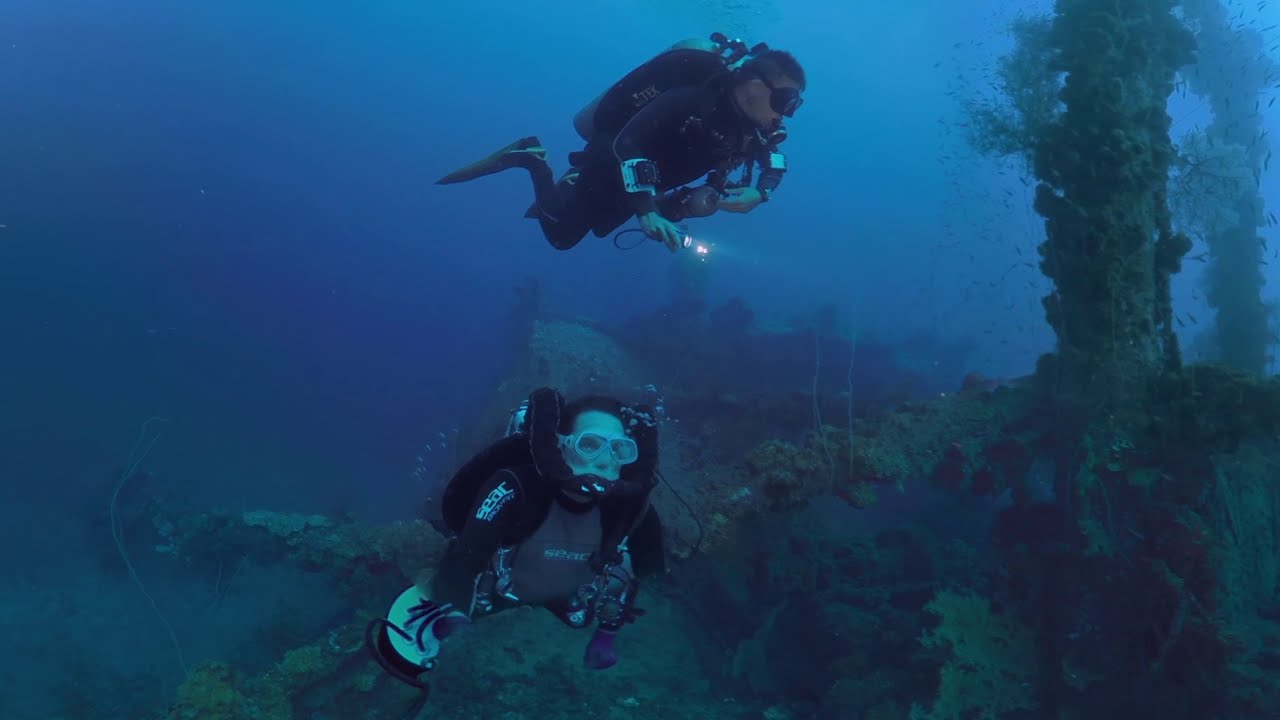The image captures a vivid underwater scene featuring two scuba divers exploring a shipwreck encrusted with vibrant marine life. Both divers, a man and a woman, are equipped with full diving gear, including wetsuits, tanks, flippers, and snorkeling masks. They each carry a flashlight, illuminating the dark blue depths of the sea. The man, positioned closer to the camera, appears to be holding a cylindrical object, while the woman explores the area above. They are surrounded by green coral and algae, which cover the ship’s mast and other protrusions, suggesting the remnants of a vessel. This underwater landscape is rich with marine flora, such as barnacles and little weeds, adding to the mysterious, adventurous ambiance of their underwater exploration.